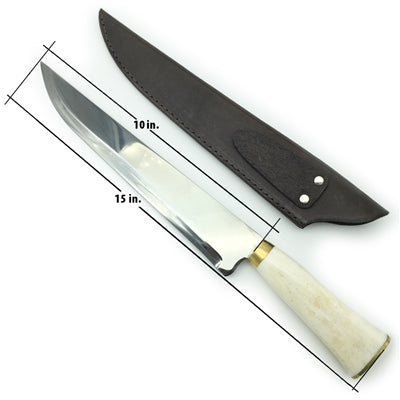The image depicts a high-quality, sturdy knife with a stainless steel blade. The knife is positioned with the tip angled toward the upper left and the ivory-colored handle extending to the lower right. The handle is accented with gold bands both near the blade and at its base. Detailed measurements show the blade is 10 inches long along its flat edge and 15 inches total, taking the curve into account. Accompanying the knife is a well-crafted, durable sheath made of brown leather. The sheath features intricate stitching and two small silver buttons as decorative elements. The overall appearance of both the knife and the sheath suggests high craftsmanship and sharpness, although no specific type or intended use for the knife is indicated.